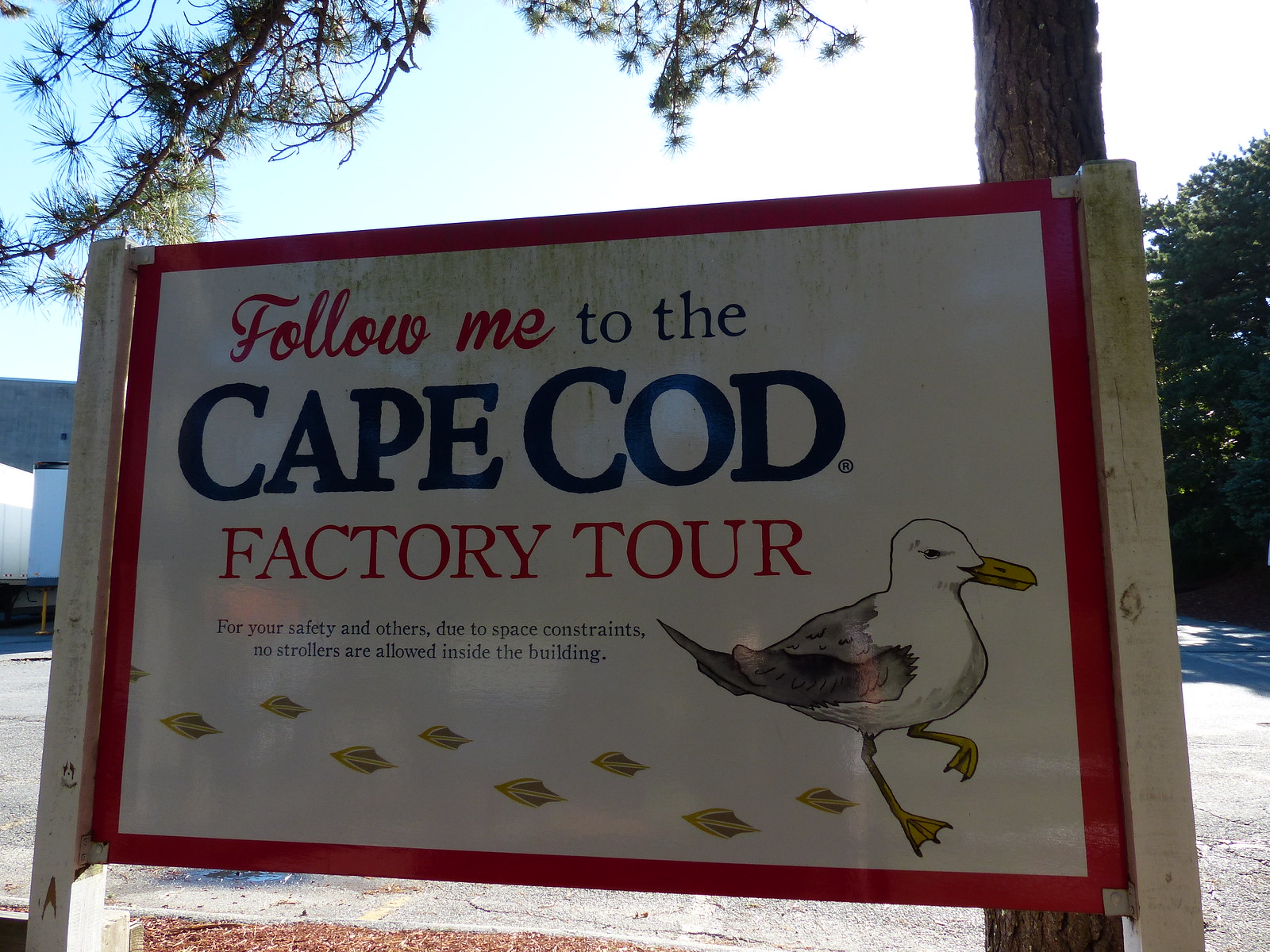This photograph captures an outdoor scene featuring a rectangular wooden sign mounted on two white posts. The sign has a red border and a light brown background. At the top left, the text “Follow me” is written in cursive red letters, followed by blue block letters instructing, “to the Cape Cod Factory tour.” Beneath this text, in large blue uppercase letters, it reads "Cape Cod," and in smaller red uppercase letters, "FACTORY TOUR." At the bottom center, smaller red letters say, “For your safety and others due to space constraints. No strollers are allowed inside the building.”

A detailed illustration of a seagull is placed at the bottom right of the sign. The seagull has a yellow beak and legs, with white feathers on its head and chest, gray wings, and it appears to be mid-step, facing to the right and leaving yellow-gold footprints behind it.

In the background, there is the trunk and some leaves of a tree, a glimpse of a low white building on the left, and a sky that transitions from white on the right to blue on the left. The ground appears to have a light color, possibly resembling snow or lightly colored pavement.